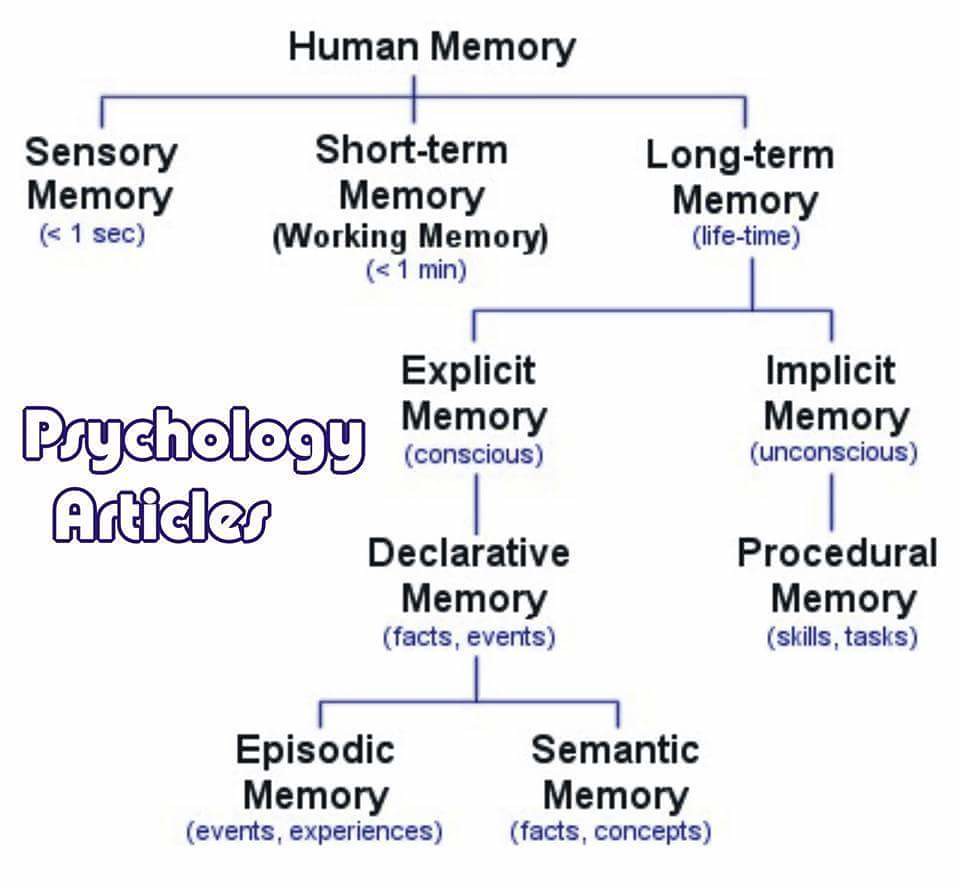The image is a detailed hierarchical chart titled "Psychology Articles," depicting the breakdown of human memory through a tree diagram. At the top, "Human Memory" branches out into three main directions: sensory memory (lasting less than one second), short-term memory or working memory (lasting less than one minute), and long-term memory (lasting a lifetime). From long-term memory, two primary branches emerge: explicit memory (conscious) and implicit memory (unconscious). Implicit memory further divides into procedural memory, which pertains to skills and tasks. Explicit memory splits into declarative memory, which is about facts and events, and this in turn branches into episodic memory (events and experiences) and semantic memory (facts and concepts). The majority of the text is written in black, while the lines connecting various elements are in blue and purple hues, emphasizing the structure of the information.